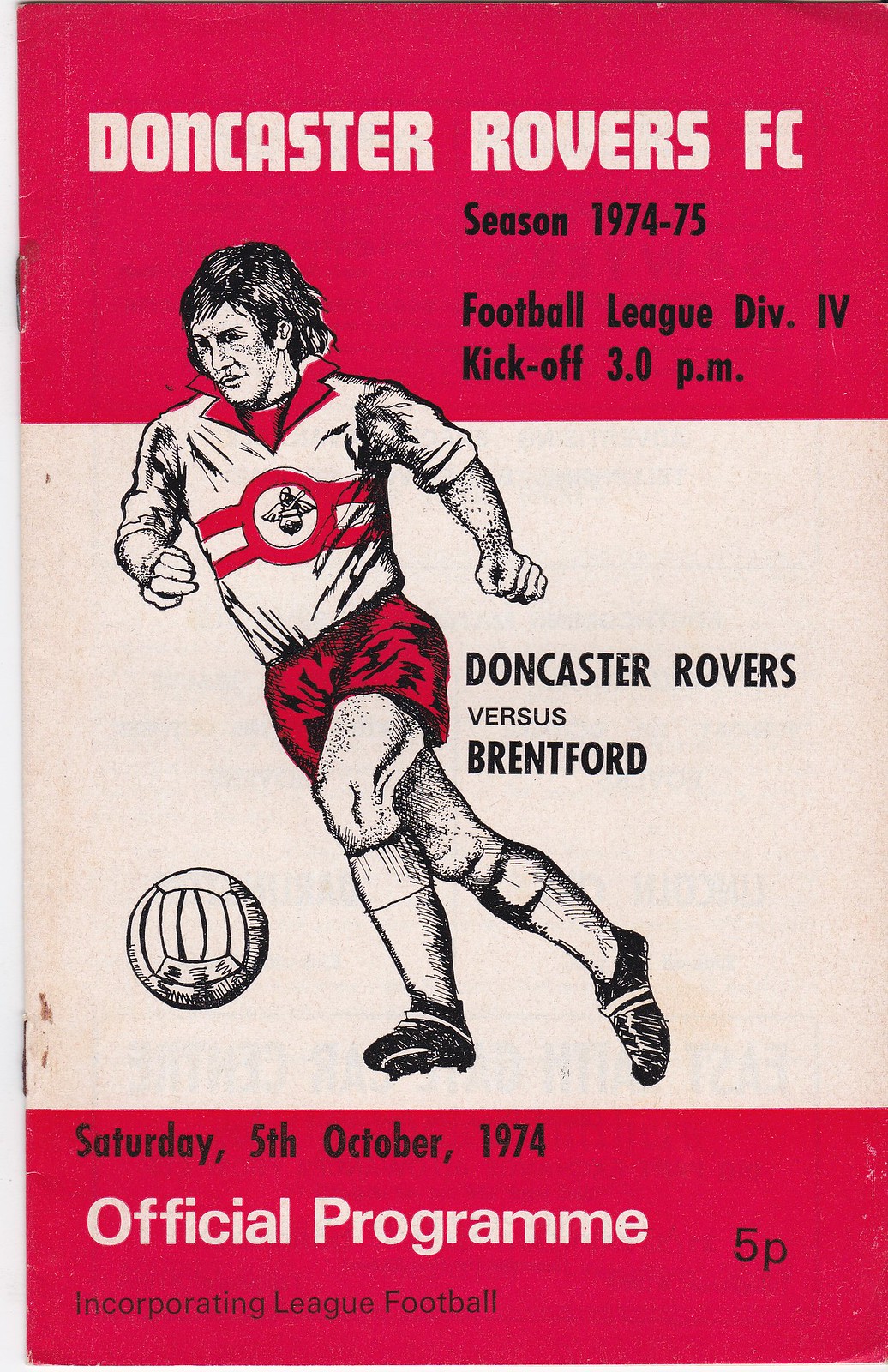The cover of the official program for Doncaster Rovers FC, dated Saturday, October 5th, 1974, is strikingly designed with a tri-color scheme. The top third is red, featuring white text that announces "Doncaster Rovers FC," and beneath it, in black text, the details "Season 1974-75, Football League Division 4, Kickoff 3 p.m." dominate. The central section is white, showcasing a hand-drawn sketch of a footballer in action, poised to kick a white soccer ball. The player is wearing a distinctive uniform: a white polo with a red collar, red shorts, white socks, black shoes, and has the Doncaster Rovers logo on his shirt. To the left of the player, it reads "Doncaster Rovers vs. Brantford" in black text. The bottom third of the cover reverts to red, with black text stating "Saturday 5th October 1974." Below this, in white text, are the words "Official Program," and to its left, black text indicates "5P" for the price of 5 pence. At the bottom, in black text, "Incorporating League Football" completes the design.